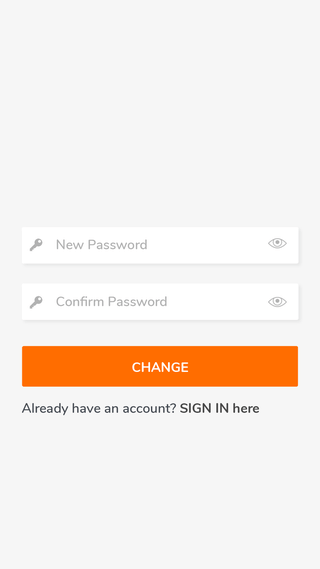The image is a screenshot of a sign-in page from a website. The visible section of the page prominently displays a form for updating a password. The first input field is labeled "New Password" and features a key icon on the left, indicating that users should enter their new password here. Additionally, there is an eyeball icon on the right, likely allowing users to toggle the visibility of their input. Below this, there is a second input field labeled "Confirm Password," also accompanied by the same key icon on the left and eyeball icon on the right, indicating that users must re-enter their new password for confirmation. At the bottom of the form is a rectangular button labeled "Change," signaling users to submit their new password information. The rest of the page appears to be either unavailable or intentionally blurred out, focusing attention solely on the password update section.